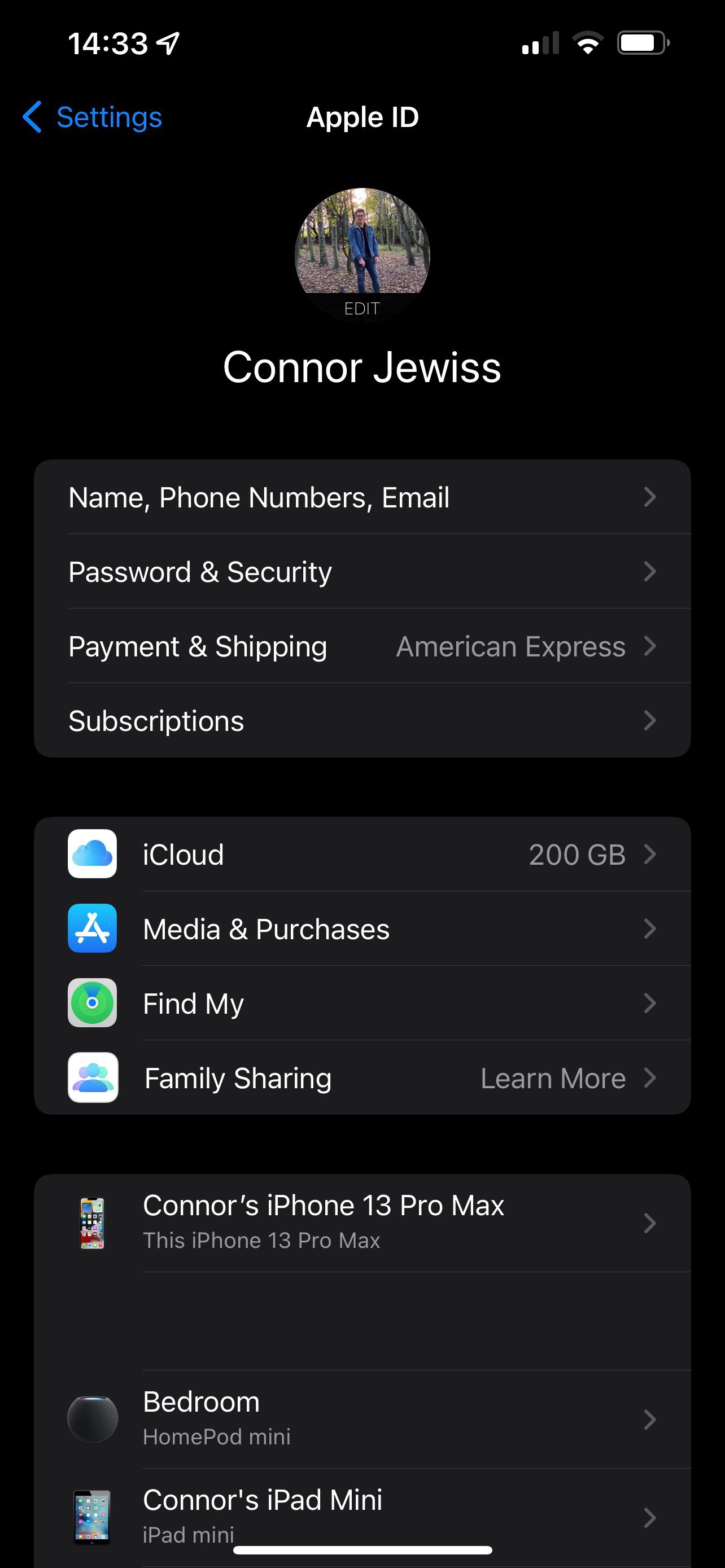The image displays a screenshot captured on an Apple device, featuring a black background typical of the device’s settings interface. At the top-left corner, beneath the time display, the word "Settings" is highlighted in blue. Adjacent to it on the right, the text "Apple ID" appears in white. Below the "Apple ID" label, there is a circular profile picture, under which the name "Conor Jowis" is prominently displayed in white text.

Beneath Conor Jowis's name, four rows list the following sections: "Name, Phone Numbers, Email," "Password and Security," "Payment and Shipping," and "Subscriptions." Each section is clearly delineated to guide the user through different aspects of their account settings.

Further down, the interface displays a series of four icons arranged vertically, each accompanied by their corresponding labels to the right. The first icon represents "iCloud," followed by icons for "Media and Purchases," "Find My," and "Family Sharing." Each icon and label is designed for easy navigation within the Apple ID settings menu, providing users with quick access to essential features and services.